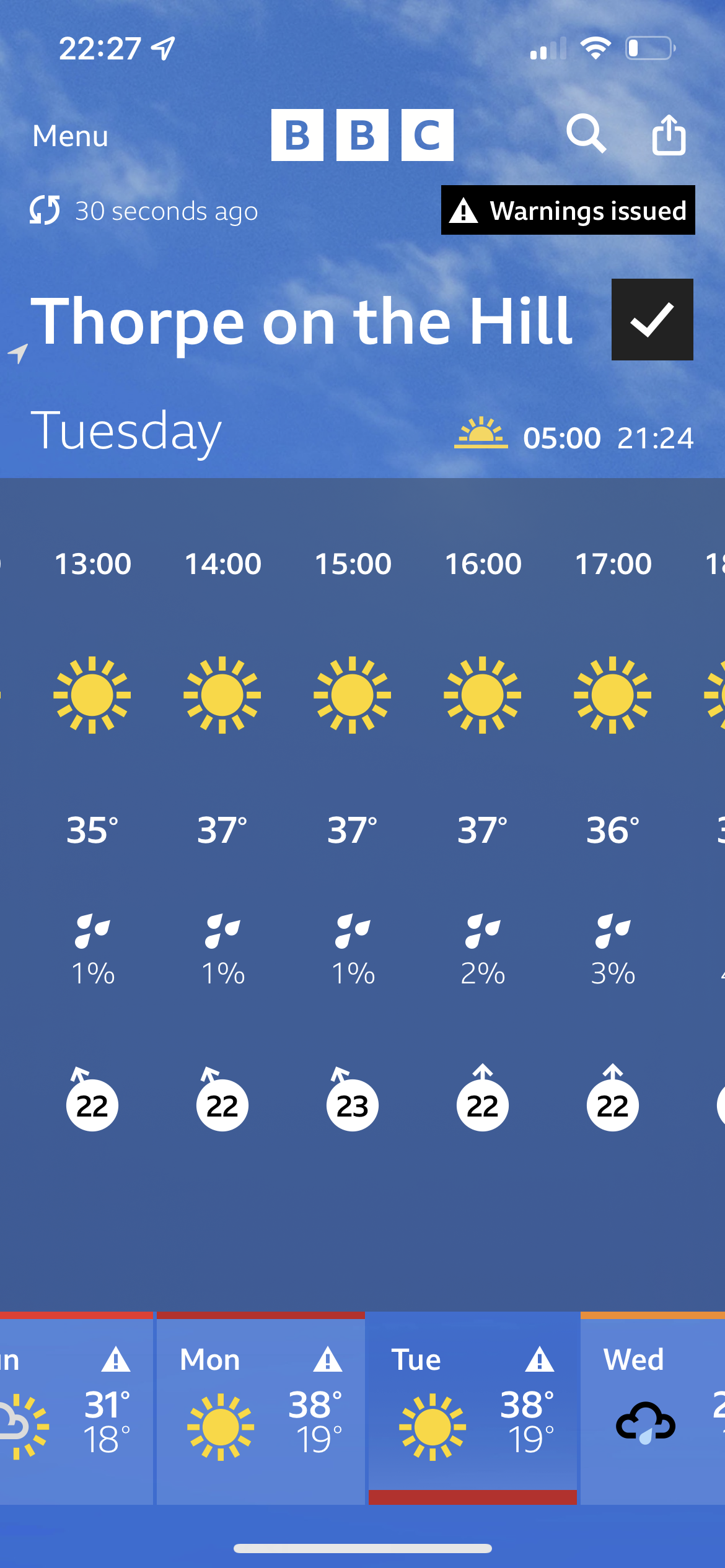This is a detailed mobile screenshot taken from a smartphone, showing pertinent weather information on a BBC branded app. The top section of the screen indicates it's from the "BBC" with a timestamp of "30 seconds ago" and a notification box declaring "Warnings Issued." Below, a bold header reads "The Rope on the Hill," with a check mark next to it. The screenshot highlights Tuesday’s date (21, 24) with a sun icon and the time "5 PM." 

The screen is filled with weather details: temperatures, humidity, and other icons denoting weather conditions across days of the week. There’s extensive data for each hour: at "1 PM," it's a sunny "35 degrees," at "2 PM," "37 degrees," and the trend continues with a slight drop in temperature towards the evening. Precipitation chances are minimal, with percentages hovering around 1-3%. Wind directions are included, enhancing the detail. The bottom of the screenshot presents a broader forecast with Monday showing a high of "38" and low of "19," while Tuesday repeats the same high and low temperatures. The interface also includes typical phone indicators like reception, Wi-Fi, battery status, a menu option, search button, share button, and navigation icons.